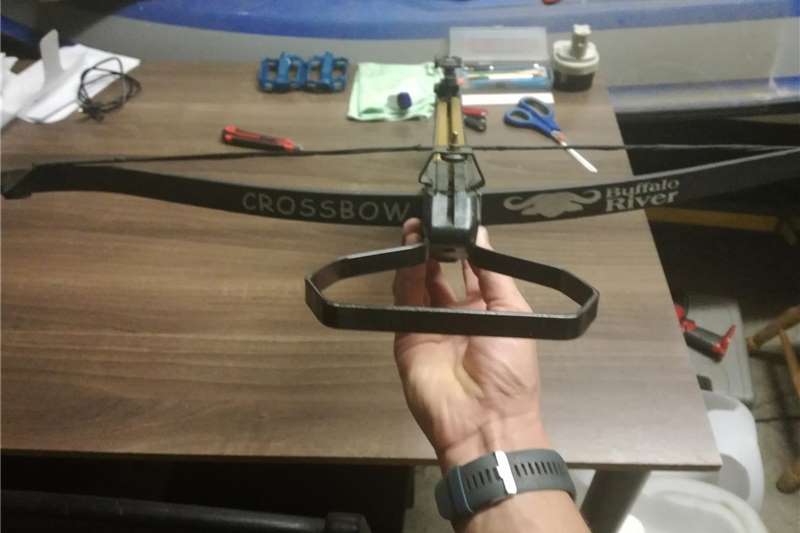In the image, a right hand with a gray wristwatch on the wrist is firmly holding a crossbow. The hand's palm is turned upward as it supports the crossbow, which is partially resting on a brown wooden table with a horizontal grain pattern. The crossbow features white lettering with the word "crossbow" on its left side, while on the right side, it displays a buffalo head logo followed by the words "Buffalo River" in white lettering.

The table surface is scattered with various items. Directly behind the crossbow, there is a pair of blue-handled scissors alongside a red-handled tool, which might be a Swiss Army knife or a screwdriver. Towards the center of the table, two blue objects resembling mixer beaters are evident. To the left, a black cable is wound into a messy ball next to a white object. Additionally, behind the blue scissors, a white and brown object stands out with a white square protruding from its top. On the floor under the table, the legs of a wooden chair are visible, and a red-handled tool with black features can be seen lying on the ground. Various documents and black USB cables are scattered across the table’s surface.